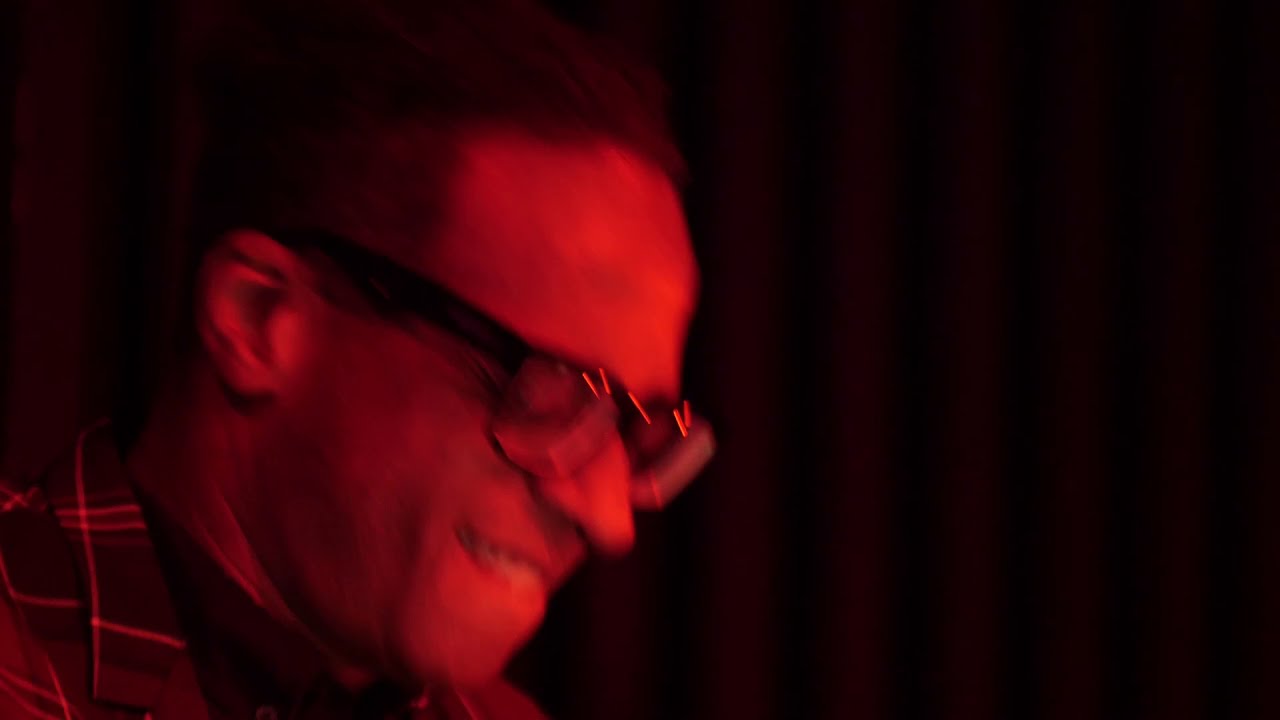In this image, we see a photograph of a middle-aged man, likely in his 40s, with darker skin and short hair. He is wearing thick, black-framed glasses and has no beard or mustache. The man's head is tilted slightly downwards and to the right as he bites his lower lip, giving the impression of a slight smile. He is dressed in a checked or plaid coat over a darker shirt. The composition primarily shows his face, neck, and a portion of his shoulders, with his eyes closed.

The background features what seems to be a dark, possibly black curtain with slight wrinkles, adding texture to the backdrop. The entire scene is bathed in a red glow, casting a reddish tint across both the subject and the background. This red lighting effect lends a somewhat blurry and dark ambiance to the overall image.